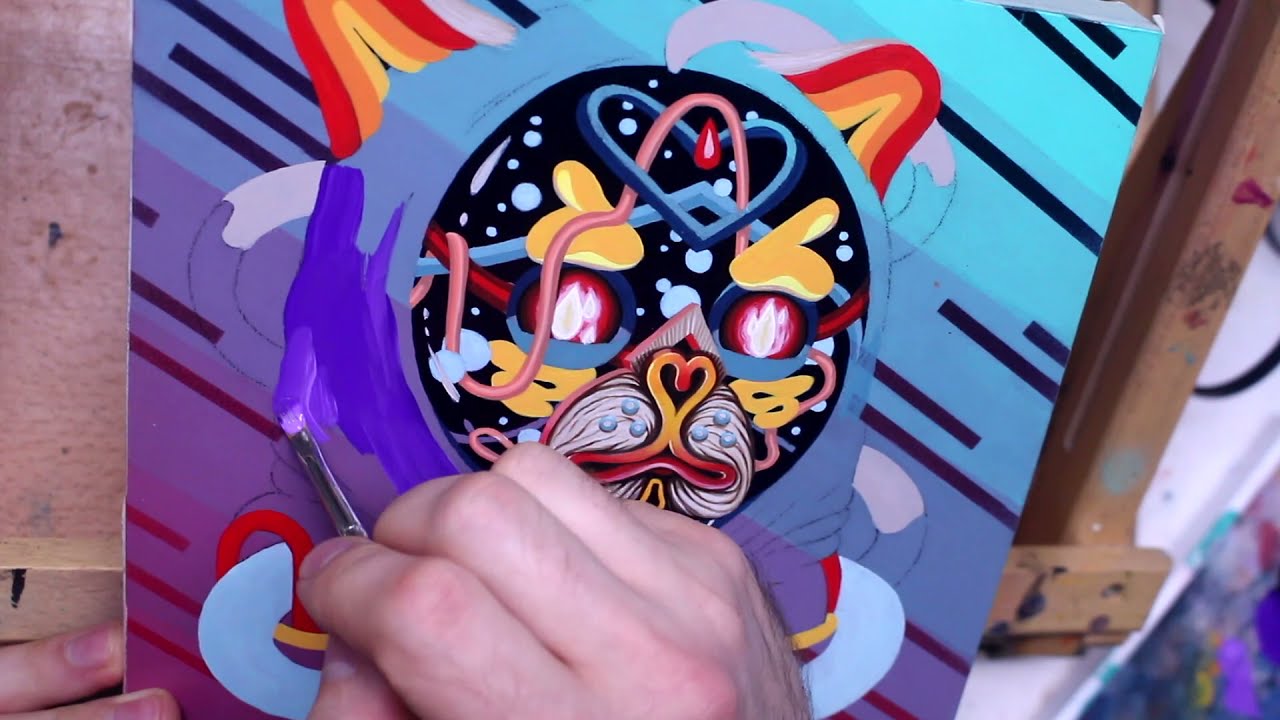A person is actively painting a vibrant, abstract image on a small canvas, held in their left hand. Their right hand wields a thin paintbrush dipped in purple pigment, applying it to the artwork. The painting features a fantastical creature reminiscent of an Ewok or a cat, characterized by its bold, colorful, and geometric design. The creature’s face is black, ornamented with round, red eyes that seem to contain either fire or drops of water. Its eyebrows are abstract, heart-shaped, and colored in yellow. The creature has striking red and yellow striped ears, while a white object surrounding its face is tinged with purple and blue. The background of the canvas transitions from light to dark shades of teal and blue, interspersed with black lines and additional colors such as green. Splashes of scattered paint in blue, yellow, orange, and purple add to the chaotic creativity of the scene. The overall setting suggests the painting could be part of a time-lapse project, with the lower half of the image revealing the artist's hand and a wooden easel partly visible in the background.